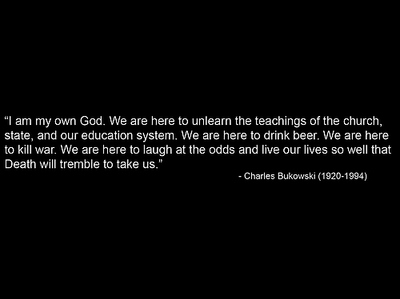A rectangular image with a solid black background features a white, center-aligned quote spanning four lines. The quote reads, "I am my own God. We are here to unlearn the teachings of the church, state and our education system. We are here to drink beer. We are here to kill war. We are here to laugh at the odds and live our lives so well that death will tremble to take us." Below the quote, in smaller white text near the bottom right corner, it states, "— Charles Bukowski (1920-1994)," attributing the quote to the renowned writer and poet.